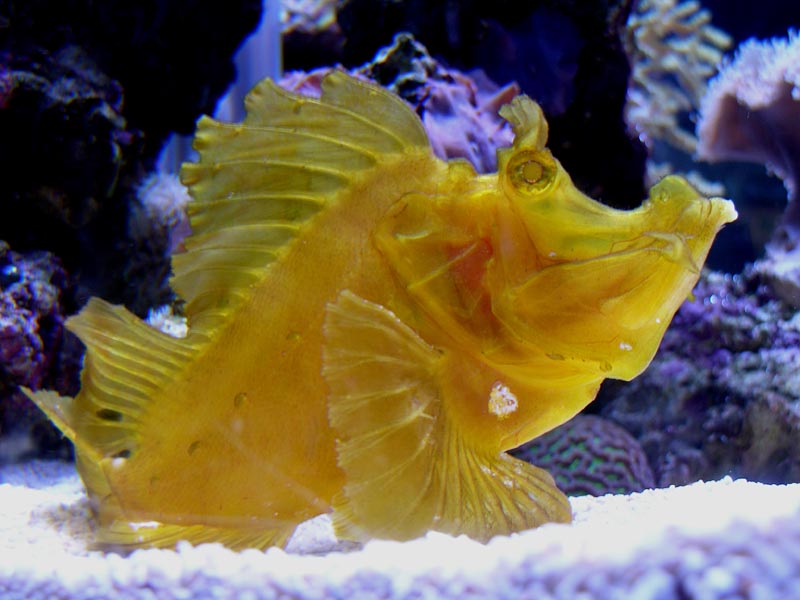This detailed photograph captures a unique fish in an aquarium setting. The fish displays a striking design, with a semi-translucent body predominantly yellow and accented with orange around its gills. Its head, shaped like an arrowhead and resembling that of a horse with a curved snout, features large yellow eyes and small yellow tendrils above them. The fish is positioned prominently in the center of the image, its side profile fully visible as it rests on a bed of fine, white gravel, possibly composed of tiny white rocks or seashells. The aquarium background is slightly blurred but shows various types of decorative coral and rocks, adding to the underwater ambiance. The photograph appears to have been taken through glass, as evidenced by a reflective hue and a reflection visible in the bottom right corner. The overall color palette includes shades of black, blue, purple, yellow, orange, and green, highlighting the vivid and intricate details of both the fish and its habitat.